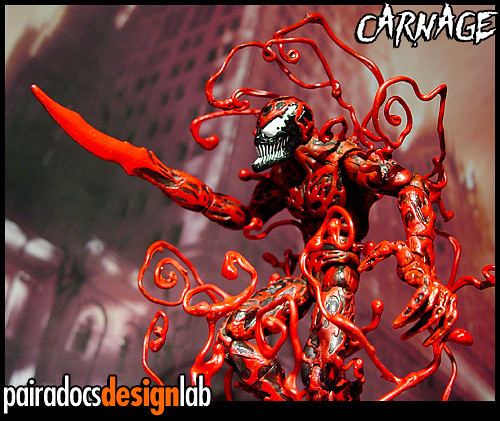This highly detailed photo captures a striking figurine of Carnage, the infamous character from the Spider-Man universe, closely associated with the Venom storyline. The figure stands against a backdrop that appears to be a rendered model of a city, viewed from a top-down angle. Carnage's menacing form is predominantly black, adorned with a vivid red, blood-like or ooze texture that seems to pulsate across his body. His large, menacing white eyes and sharp white teeth jut out from his elongated mouth, adding to his haunting appearance.

Carnage's chaotic form is further accentuated by the red tendrils or tentacles that extend from his arms, back, and legs. His right arm morphs into a grotesque red blade, while his left arm, positioned near the bottom right side of the frame, is an open clawed hand ready to grasp. The red lines and squiggles of his oozing substance give the impression of life and movement, akin to the symbiotic nature of the characters in the Venom series.

In the top right corner, "Carnage" is emblazoned in white letters against a black outline, asserting the figure's identity. The bottom left corner proudly identifies the creators with the text "Paradox Design Lab," featuring 'Design' in eye-catching orange, and the rest in white with a contrasting black outline. This meticulously crafted piece, possibly made of clay or a similar material, captures the chaos and ferocity of Carnage, making it a fascinating and dynamic representation of this iconic villain.